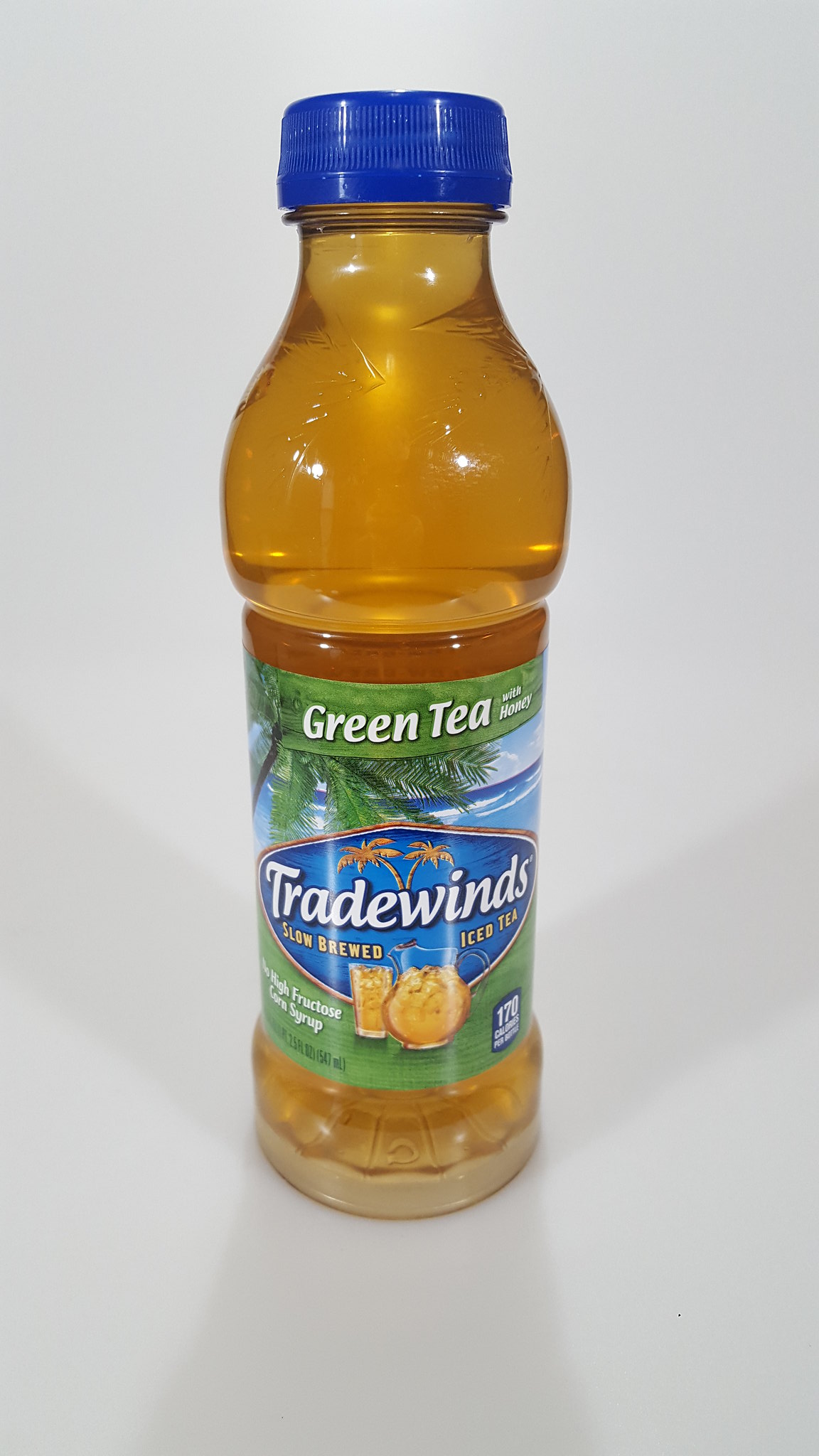This is a vibrant color photograph depicting a close-up of a single-serving bottle of tea. The bottle, which appears to be made of either glass or plastic, features a striking royal blue cap and a clear body, revealing the light brownish-amber hue of the tea inside. At the top of the bottle, a colorful label prominently displays the words "Green Tea." The background evokes a natural theme with the image of a tree intertwined in the design. The label includes a blue oval, serving as a base for the "Trade Winds" logo, written in bold lettering. Below the logo, an illustration of a glass of tea alongside a clear glass pitcher filled with iced tea adds a picturesque touch. The label even has some gold writing, although it is too small to decipher in this photograph.